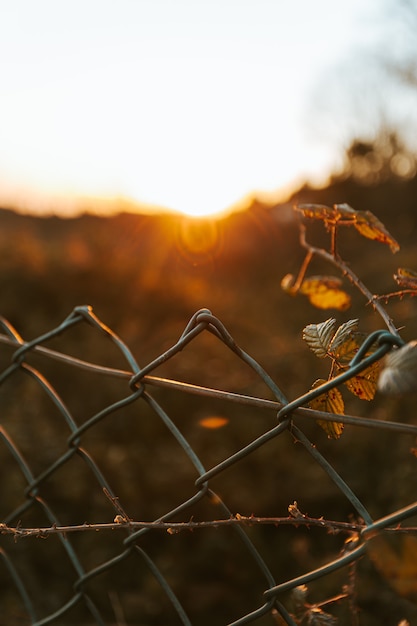The photograph captures the top of a barbed wire fence arranged in diamond shapes, with thin branches or twigs from a bush intertwined through portions of the wire. The entire scene is bathed in a warm, orange hue, likely due to the setting sun casting a yellowish-orange glow across the frame. In the background, the horizon is visible with the backlight making the sky appear mostly white, though it seems to transition to a light blue towards the right side. A few leaves can be seen growing on the intertwined branches, adding a touch of greenery to the composition. The wire fence itself appears slightly rusted, emphasizing its weathered state amidst the glow of either sunrise or sunset.